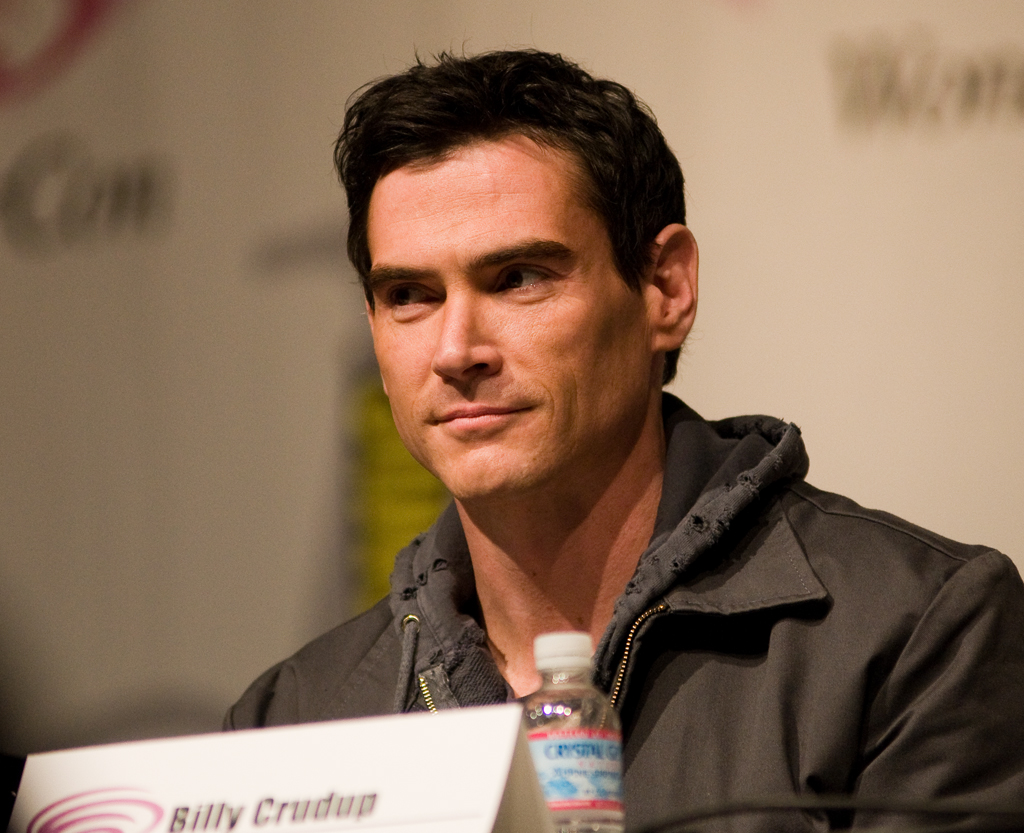In this photograph, Billy Crudup, a white male with dark hair, is seated at a table, likely at a press conference or a convention like Comic-Con. He is wearing a layered outfit comprising a gray, hole-speckled hoodie and a deep greenish-gray zip-up jacket with drawstrings. In front of him on the table, there's a bottle of water and a white paper nameplate that reads "Billy Crudup." He is looking off into the distance with a slight smile on his face, suggesting engagement with the audience. Behind him, the backdrop features a white wall with out-of-focus black letters and a yellow graphic, likely representing the logos of event sponsors.